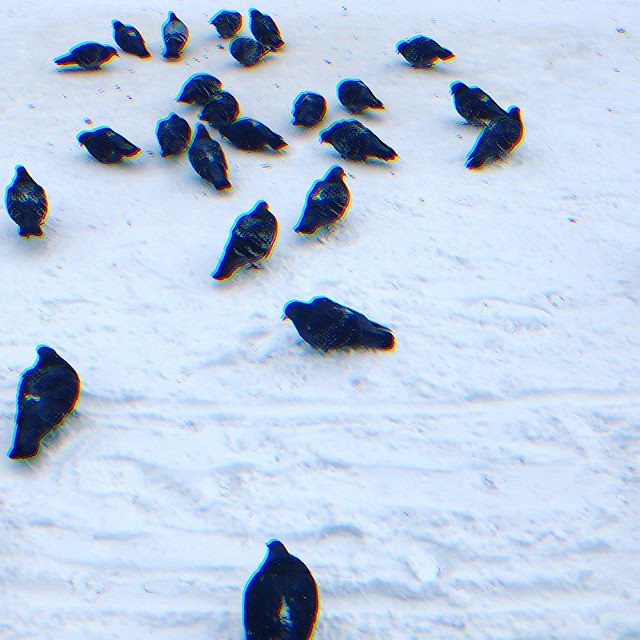The image captures a mesmerizing scene of a large group of around 25 blackbirds or crows standing and moving about on a snowy landscape. The snow appears soft and powdery, featuring subtle hills and indents that add texture to the white background. The picture has a trippy, abstract feel to it, with grainy effects and wavy colors—hues of blue and red—that outline the birds, creating a sense of motion and depth. Some birds are closely packed at the top of the photo, while a few are scattered towards the bottom. The image also includes black marks suggesting weathering or wear, adding to the overall ethereal quality of the scene.